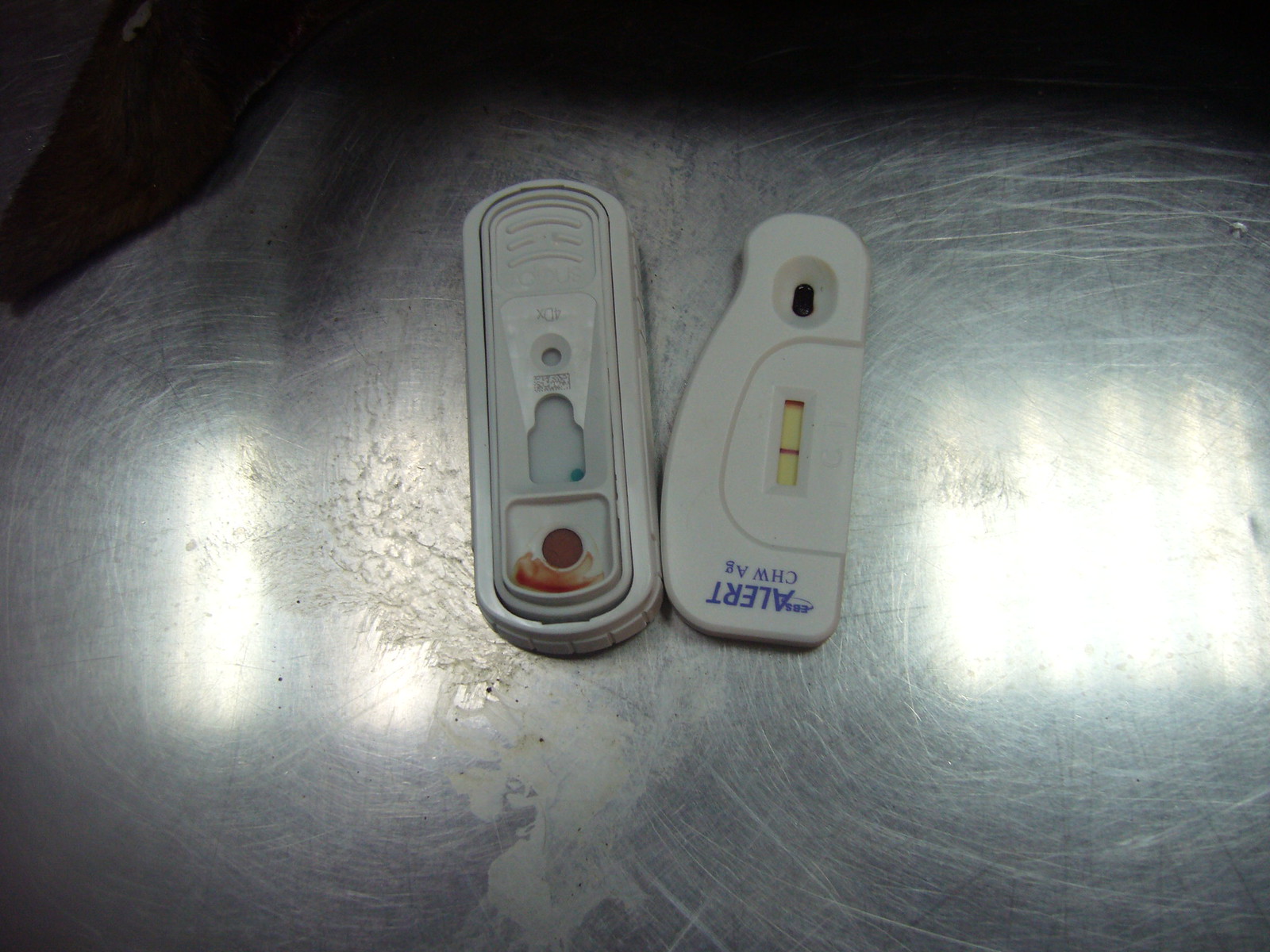This photo captures a testing device in landscape orientation from an overhead perspective. The image showcases two distinct pieces, potentially components of the same device, placed side by side and touching. The piece on the right, likely a lid or top, is displayed upside down, revealing the lettering "ALERT CHWAG." The purpose or meaning of this text is unclear. The piece on the left appears to be the bottom or base and contains a visible pool of blood, obscuring its function or the specifics of what it is testing. Both objects are set on a well-worn and slightly dirty aluminum surface, akin to a commercial kitchen counter made of stainless steel. The surface is marked by numerous scuffs and scratches. The close-up nature of the photograph highlights the dull reflection of lights on both sides of the objects, with no other elements visible in the frame.